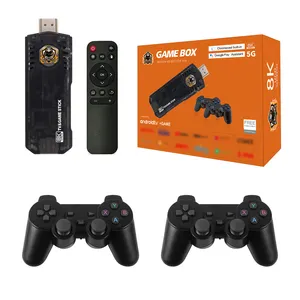This image is a detailed product display for a video game system boxed in orange packaging labeled "Gamebox" in white on the upper right corner. The prominently featured orange box has "8K" and "Gamebox" written on it in white lettering and is set against a white background. Surrounding the box are four pieces of equipment: a TV game stick shaped like a larger zip drive, a streamlined remote control with a red button in the top left corner and black buttons with directional arrows, and two wireless game controllers reminiscent of PlayStation 3 controllers. The controllers are black and have dual thumbsticks resembling joysticks, directional arrow keys on the left, and various control buttons with labels including "X" on the right.